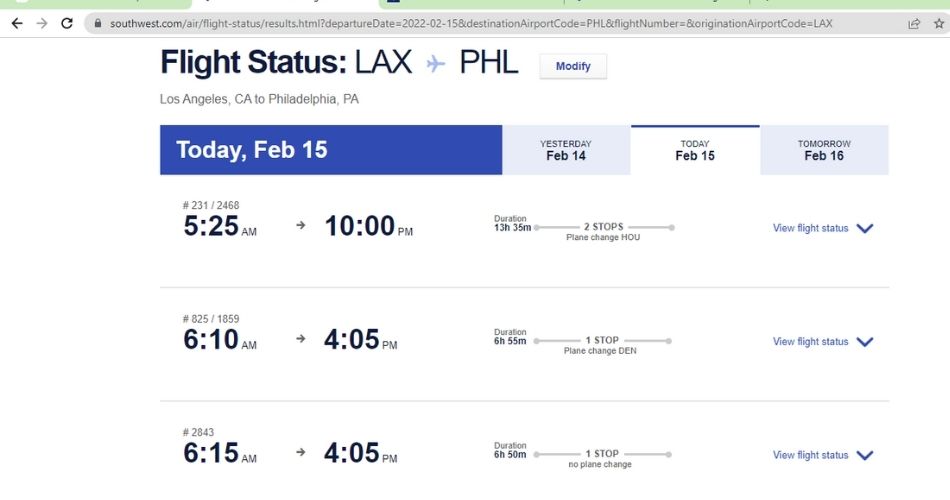**Screenshot of Flight Status Page on a Travel Website**

The image depicts a screenshot from a flight status page on a travel website. At the very top, there is a thick, light green horizontal line followed by a white section and then another thick light green line. Below this, there's a banner featuring navigation buttons: a left arrow key, a right arrow key (muted out), a refresh icon, and a light gray address bar displaying a website address.

In the white section beneath the address bar, the title "Flight Status" is displayed prominently in bold, capitalized text with the letters "F" and "S" capitalized. Following the title is a colon, then the text "LAX to PHL," indicating a flight from Los Angeles International Airport to Philadelphia International Airport. To the right, a blue rectangular button with the word "Modify" in white text can be seen, providing an option to adjust the search criteria.

Further down, the text "Los Angeles, California to Philadelphia, PA" is displayed, and beneath it, a blue banner highlights the text "Today February 15th" in white. Adjacent to this are options for "Yesterday February 14th" and "Tomorrow February 16th".

The image further lists the details of multiple flights:
1. **Flight 1:** 
   - Time: 5:25 a.m. to 10:00 p.m. 
   - Duration: 13 hours 35 minutes 
   - Stops: 2 
   - Plane change in Houston

2. **Flight 2:** 
   - Time: 6:10 a.m. to 4:05 p.m. 
   - Duration: 6 hours 55 minutes 
   - Stops: 1 
   - No plane change mentioned

3. **Flight 3:** 
   - Time: 6:15 a.m. to 4:05 p.m. 
   - Duration: 6 hours 50 minutes 
   - Stops: 1 
   - No plane change

The details are presented in a structured manner, providing clear and accessible information regarding flight options from Los Angeles, CA to Philadelphia, PA.